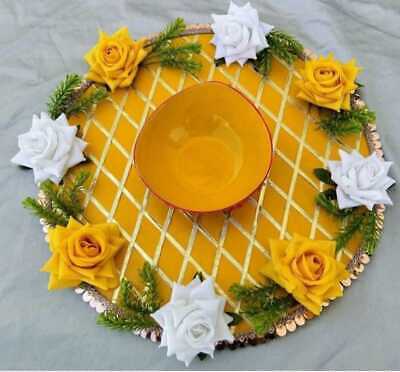The image features a detailed and intricately arranged art piece set against a white fabric backdrop. Central to the composition is a vibrant orange ceramic bowl with a thin red rim, giving it a polished appearance. This bowl rests on a flat, circular base adorned with a crisscross pattern of white or possibly silver lines cutting across a yellow background, creating a series of yellow diamonds. Encircling the base, an alternating arrangement of yellow and white roses is interspersed with sprigs of green pine needles for added texture and visual interest. Additionally, small circular accents in silver, gold, and black are found around the outer edge of the base, enhancing the decorative quality of the piece. The overall presentation is brightly lit, emphasizing the clarity and vivid colors of the arrangement.